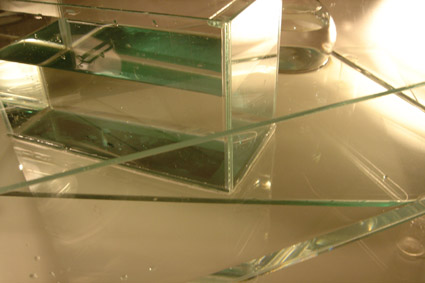In this image, a rectangular glass container is prominently featured. The container is relatively small and segmented into several shelves. Most of these shelves are empty, but the top shelf holds a solitary paper clip. This glass container is positioned on a transparent glass shelf, which itself is part of a larger shelving unit with a metallic border enclosing the shelf below. Adjacent to the glass container is a small, round, clear structure that resembles a vase or tumbler. The scene is accentuated by the clean, minimalist design and the interplay of glass and metallic elements.